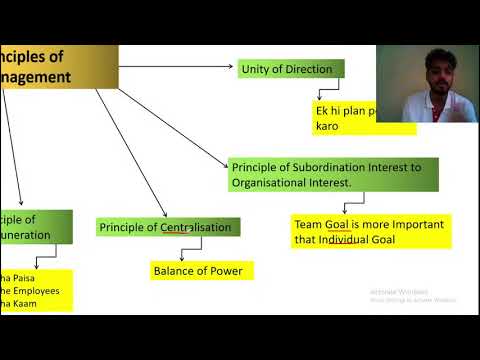The image portrays a PowerPoint slide presented during a video call. The main screen is dominated by a white slide featuring a detailed flowchart. In the upper right-hand corner, there is a small thumbnail image of a man with short black hair, a tan face, and a black mustache, dressed in a white shirt, who appears to be addressing the webcam, likely the presenter.

The flowchart begins with a central gold-colored rectangle in the top left corner, labeled "Principles of Management," though some of the text is cut off. Arrows stem from this box, leading to several green and yellow boxes. Key concepts in these boxes include "Principle of Centralization," "Principle of Subordination Interest to Organizational Interest," "Unity of Direction," and "Balance of Power." Below these, additional yellow rectangles feature further details such as "Team Goal is more important than Individual Goal" and text in another language. The lower part of the flowchart includes a box with the phrase "Simple of Uneration and Employees." The slide is framed by black borders at the top and bottom, providing a structured layout for the information being presented.